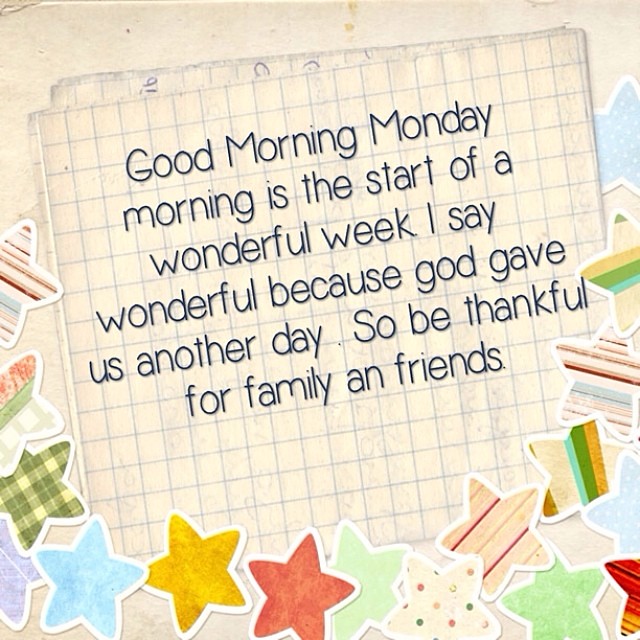This image appears to be a digitally crafted greeting card or inspirational poster, designed with a textured beige background that resembles sandy tan paper. Stylishly overlaid in the center is an angled notepad or graph paper adorned with a heartfelt message reading: "Good morning Monday. Morning is the start of a wonderful week. I say wonderful because God gave us another day, so be thankful for family and friends." Surrounding the bottom of the image and creeping up the sides are numerous colorful stars, each boasting unique patterns such as plaid, sprinkles, checks, and more, adding a playful touch to the design. The text is centered prominently, though it may read like a run-on sentence due to the lack of clear punctuation. Overall, the image seems slightly blurry, as if photographed, and exudes a friendly, uplifting vibe suitable for sharing online to inspire gratitude and positivity.